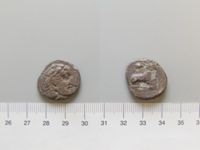The image showcases two ancient coin-like stones with etched patterns, placed slightly off-center on a white to gray backdrop. These small, silver artifacts display telltale signs of age, with irregular, hammered shapes. The left stone, appearing between the 27.5 and 29.5 cm marks on an included ruler, features a design with subtle, differing marks, suggestive of a worn face with a war helmet on one side. The right stone, located between the 32.5 and 34.25 cm marks, shows a protruding design resembling a mountain. The numeric markers on the ruler range from 26 to 36 cm, confirming this is a meticulous photographic documentation likely intended for exhibition or scholarly analysis.